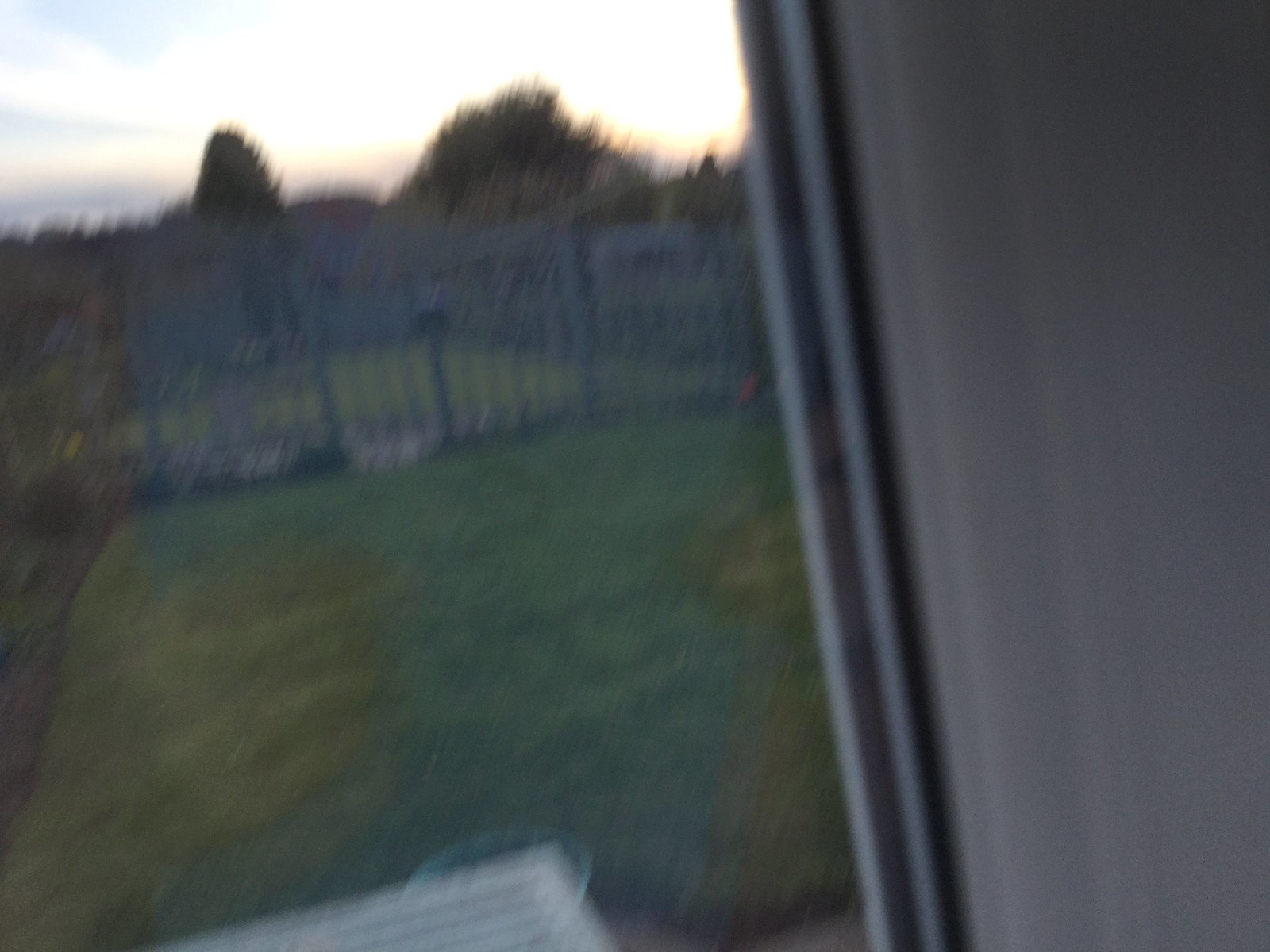Captured from inside a home, this image showcases a picturesque backyard through what appears to be a sliding glass door. A faint reflection of the photographer is visible on the glass. The yard features a line of trees in the background, and it's either early morning or early evening as the sun is rising or setting on the right side, casting an orange glow through the tree line. The sky has a grayish-white hue with hints of warm colors. The yard itself is well-maintained, with neatly trimmed grass and a black iron fence enclosing the area. There is an opening in the fence, possibly leading to a dog pen. On the right side of the image, part of the interior wall or curtain is visible, colored in light gray.